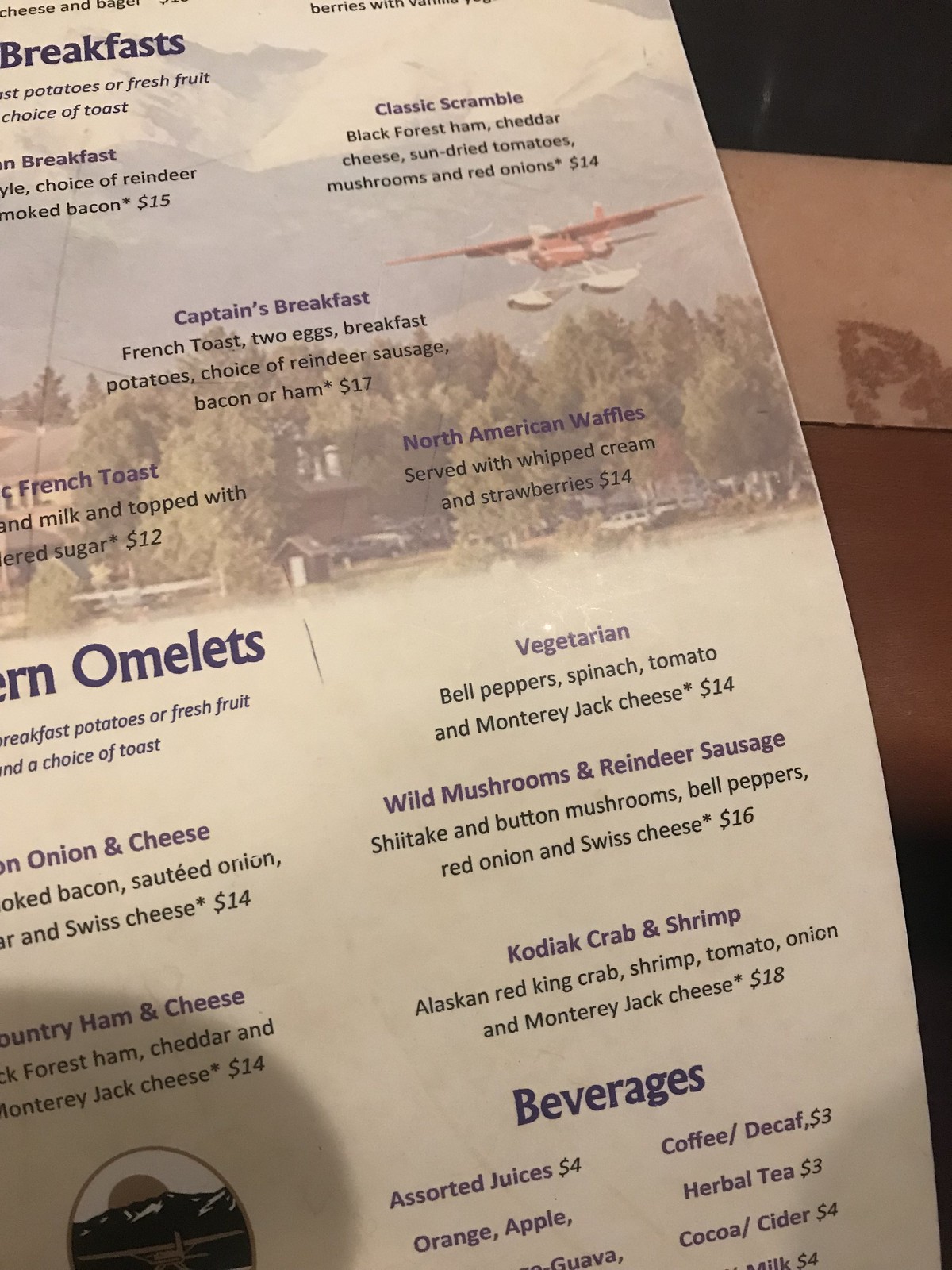The photo captures a breakfast menu placed on a table, subtly revealing the tabletop and perhaps a partial view of a placemat beneath it. The menu is organized meticulously: the top section lists various breakfast meal options, followed by a middle section dedicated to a variety of omelets, and beverages are noted at the bottom. The omelet section features intriguing combinations such as a vegetarian omelet with bell peppers, spinach, tomato, and Monterey Jack cheese, a wild mushroom and reindeer sausage omelet, and a luxurious Kodiak crab and shrimp omelet. The prices for these dishes, along with the cost of beverages and eggs, are clearly indicated. The restaurant appears to specialize in breakfast, perhaps hinting at separate menus for different times of the day. The photo, though straightforward, provides a glimpse into the thoughtful layout and rich offerings of this breakfast menu. Further context from the surrounding table or placemat remains blurred, leaving the menu as the primary focus of the image.